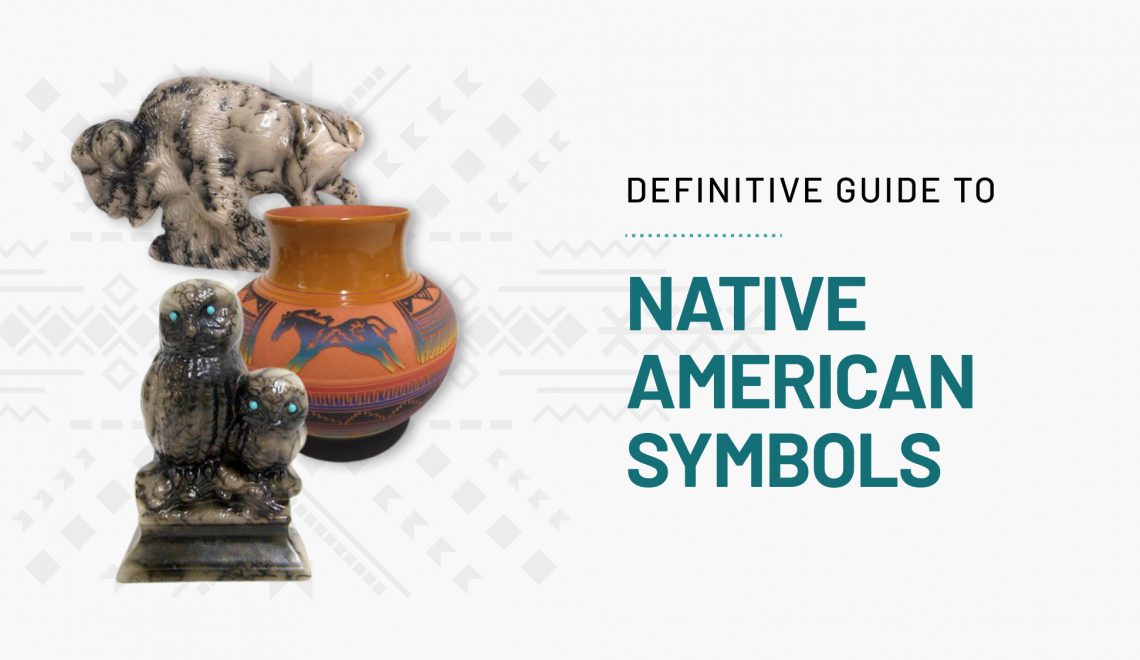This image appears to be the cover slide for a PowerPoint presentation titled "Definitive Guide to Native American Symbols." The overall background is off-white with geometric patterns in very light grey. On the right-hand side, in bold black lettering, it reads "Definitive Guide To." Below this, in a sequence of teal dots transitioning to darker blue-green capital letters, it states "Native American Symbols" over three lines. 

The left side of the image prominently features three porcelain or ceramic artifacts. In the foreground is a statue depicting two owls - one larger and one smaller - crafted in a variegated brown material with striking turquoise eyes. Behind this statue is an orange, burnt-colored vase adorned with a teal silhouette of a horse. The third item is a white buffalo statue, distinguished by black indents highlighting its detailed features and lines. The composition and artifacts suggest a thematic representation of Native American cultural symbols.